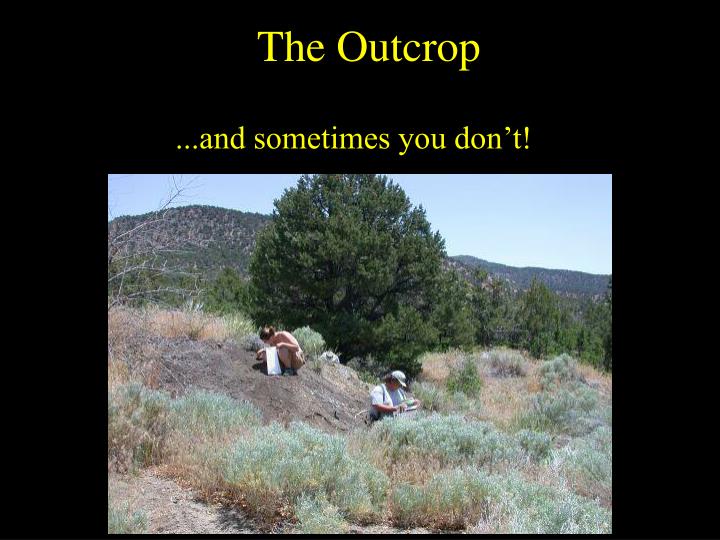The image features a black background with bold yellow text at the top that reads, "The outcrop..." followed by, "and sometimes you don't!" In the center of the image is a rectangular photo depicting a man and a woman in an outdoor, wilderness setting during daytime. They are positioned in front of a tree, which stands prominently at the middle of the image. Both individuals appear to be engaged in some form of close inspection or search; the woman, dressed in an apricot-colored top, is crouched down holding a plastic bag, seemingly picking up or examining something from the ground, while the man, who is wearing a hat and a white shirt, is looking at something he is holding. The landscape around them includes tall grass, bushes, and a mountainous background partially covered with trees.